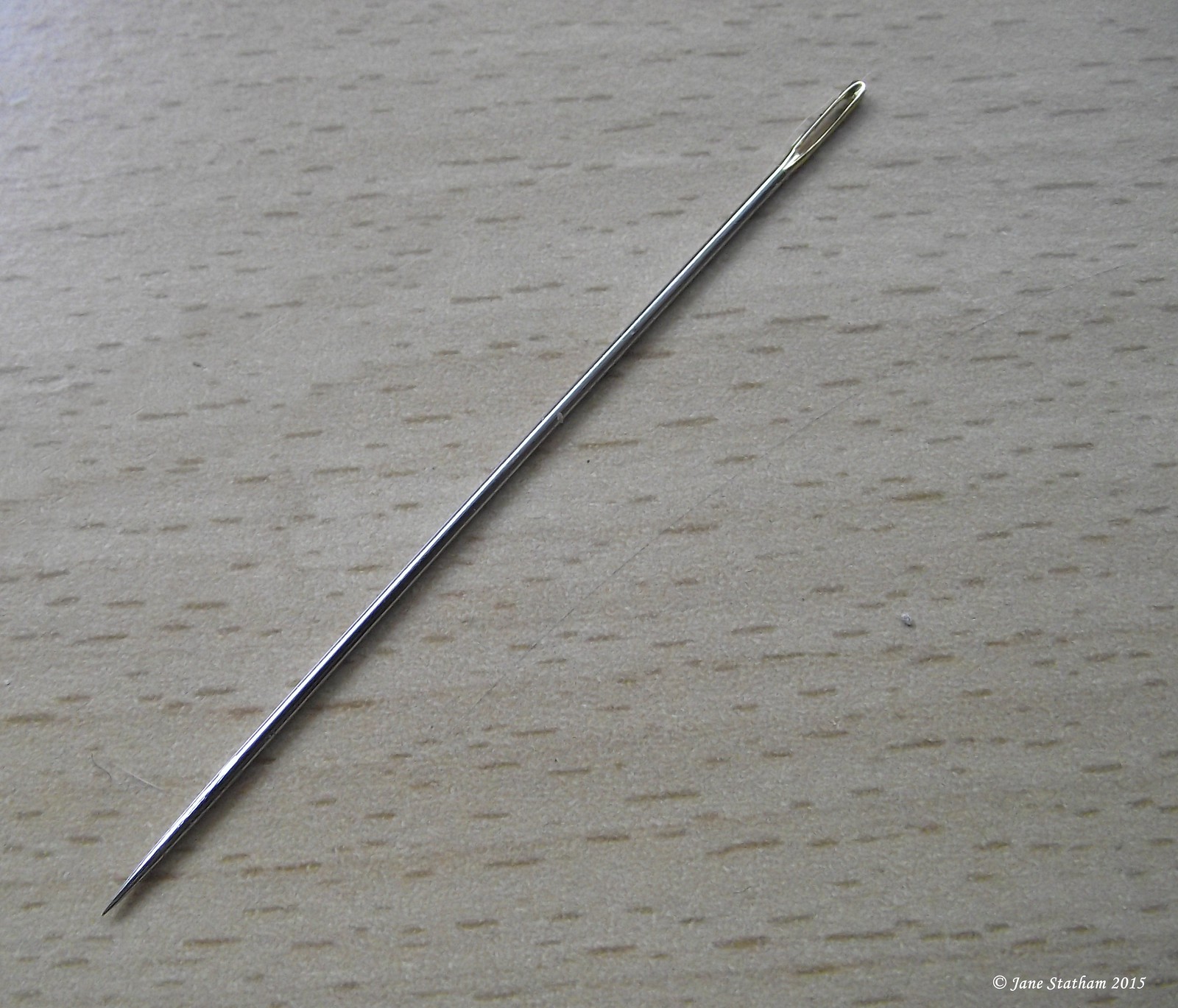The image is a close-up of a solitary metal sewing needle angled from the left to the right against a non-wood, likely laminate or Formica, table surface that has a grayish-brown color with horizontal lines. The sewing needle, made of stainless steel, appears very sharp with a pointed tip and a large elliptical hole for threading. Additionally, there are some visible hairs or scratches, indicating the image is highly zoomed in, highlighting also some smudges on the needle. The photograph is watermarked with white text at the bottom right corner, reading "Copyright Jane Statham, 2015," indicating the photographer's name and the year the image was taken.